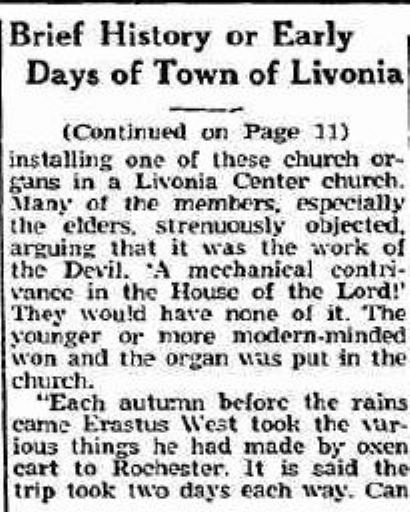The image depicts a vertical, rectangular newspaper clipping set against a white background. The clipping is bordered by a thin black line that frames the top and left sides, extending slightly down the right side as well. The text is presented in black horizontal rows. At the center-top of the clipping, bold and prominent, is the headline: "Brief History or Early Days of Town of Livonia," followed by "(Continued on page 11)." The article describes a historical event involving the installation of a church organ in a Livonia center church. Many of the church elders strongly opposed this, deeming it a devilish mechanical contrivance unsuitable for the house of the Lord, while the younger, more progressive members supported it, leading to the organ's eventual installation. The article also recounts how each autumn, before the rainy season, Erastus West would transport various crafted items by oxen cart to Rochester, a journey said to take two days each way. The clipping concludes abruptly with the word "can."